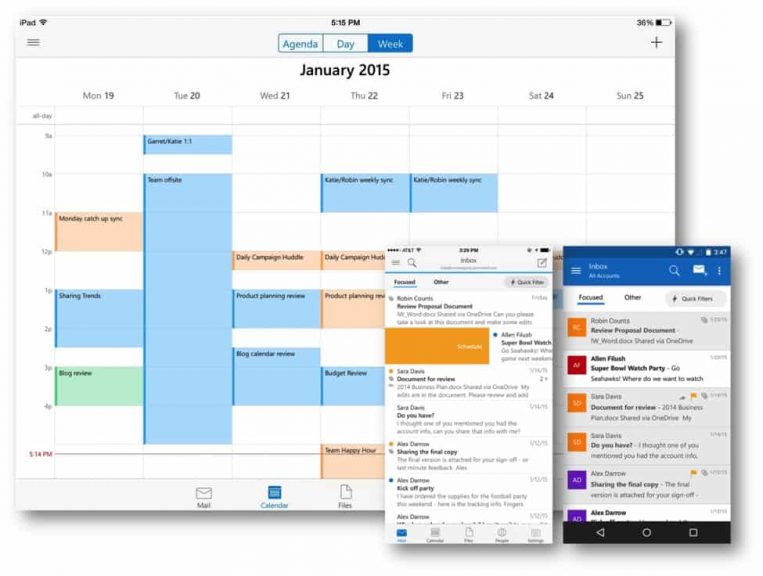The image displays a screenshot from an iPad's calendar application, captured on January 15, at 5:15 p.m. The device's battery level is at 36%, partially filled with a black indicator and predominantly white showing the remaining capacity. At the top of the screen, navigational options "Agenda," "Day," and "Week" are visible, with "Week" highlighted in a blue rectangle with white text, while "Agenda" and "Day" are simply in blue text.

The main calendar area for January 2015 illustrates various scheduled events. Events are color-coded: light blue, orange, and green, representing different categories or priorities. Additionally, two overlay windows appear on the screen, resembling pop-up notifications or additional interface elements; one labeled "Schedule" and another "Inbox," suggesting interactive options for managing tasks or messages.